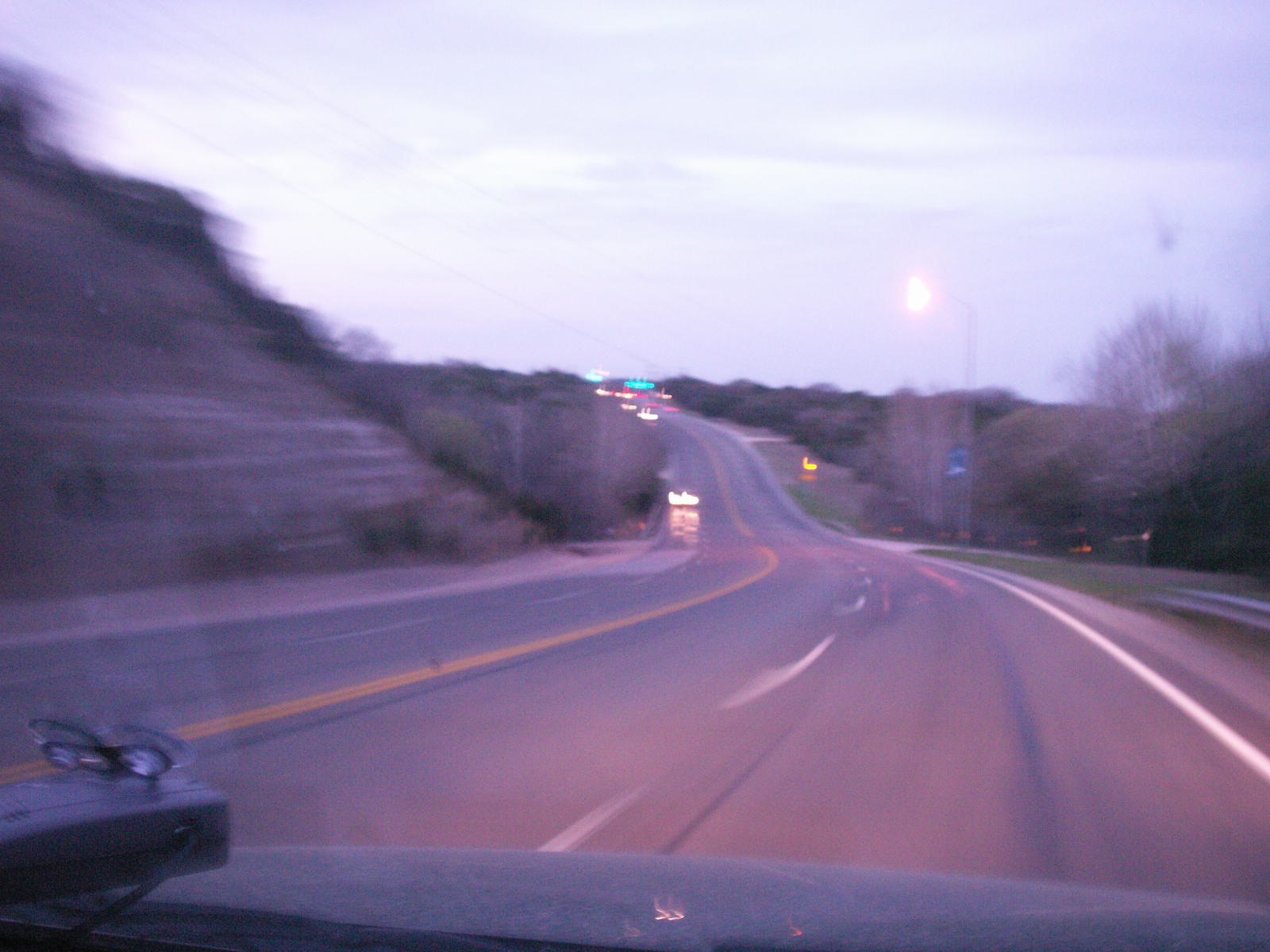This image captures a dynamic moment inside a moving car, viewed from the passenger seat. The dark-colored vehicle's hood and dusty dashboard are visible, along with a black rectangular device, possibly a dash cam, suction-cupped to the windshield. The scene outside the windshield is of a slightly winding two-lane highway set against a backdrop of a lightly cloudy sky with patches of blue peeking through, likely during dusk. On both sides of the highway, which features a solid yellow line and dotted white lines, there are trees and varying natural elements, including a rock cut with trees and grass on the left, and mounds of brown dirt with green trees on the right. A guardrail on the right is partially visible, along with a tall streetlamp. The road extends into the distance, where traffic lights glow green and the distant lights of cars—red taillights and white headlights—can be seen, indicating a traffic stop further down. Despite the motion blur in the image, the scene conveys a sense of speed and the approaching twilight hour.